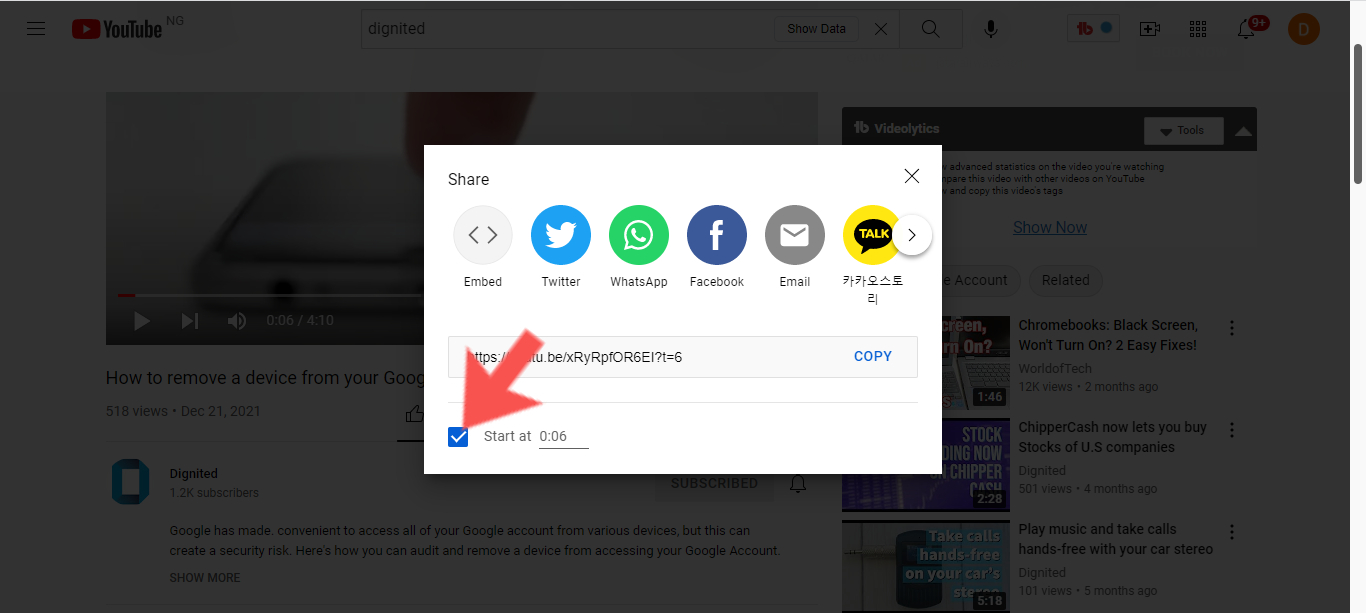The image showcases a centered pop-up window against a dimly lit, blurry background of a YouTube screen. The pop-up, with a white background, displays the word "Share" at the top left corner and an 'X' for closing on the top right. Underneath, there are five gray circular icons with arrows, each representing platforms for sharing: Twitter, WhatsApp, Facebook, and Email. A yellow circle labeled "Talk" is also present among these icons. 

Beneath these sharing options, there is a link accompanied by a blue "Copy" button on the right side. Further below is a thick red arrow pointing to a blue checkbox labeled "Start at 0:06," which is currently checked.

The dim background reveals a blurred YouTube interface, featuring a video player on the left, with comments below it, and suggested videos on the right. Standard YouTube icons are visible at the top of the screen, and the YouTube logo is situated in the top left corner of the webpage.